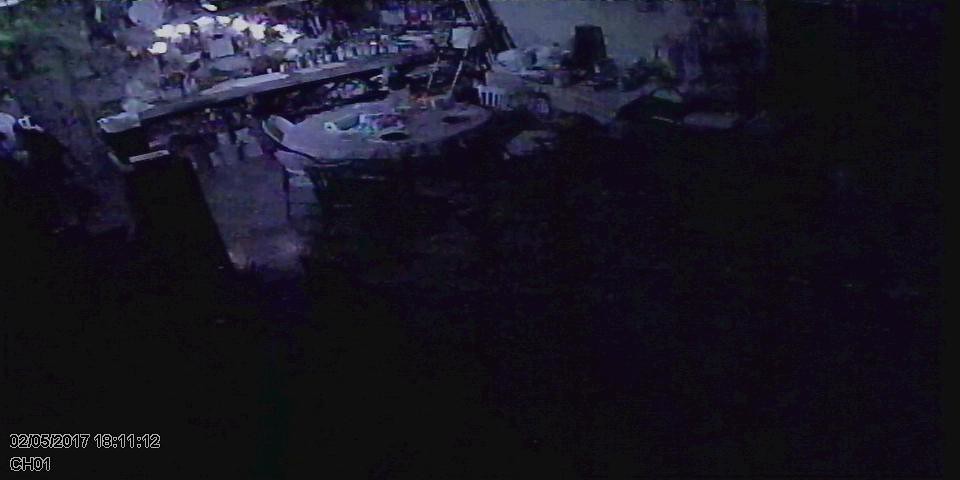The image is a wide and dark scene, predominantly black in the bottom right diagonal half. The upper left of the image possesses a dark purplish hue. In the bottom left-hand corner, a timestamp reads "02-05-2017 18:11:12," and beneath it, "ch01" indicates the channel. 

In the upper left part of the picture, a large circular table surrounded by chairs is visible, with various objects scattered around. To the right of this circular table, there appears to be a long table. Further up to the left, there is a series of tables or a single long, thin rectangular table, flanked by an array of lights above. In the very upper left corner, what seems to be the tops of trees are faintly discernible. The image evokes an evening atmosphere, potentially resembling a computer-rendered scene.